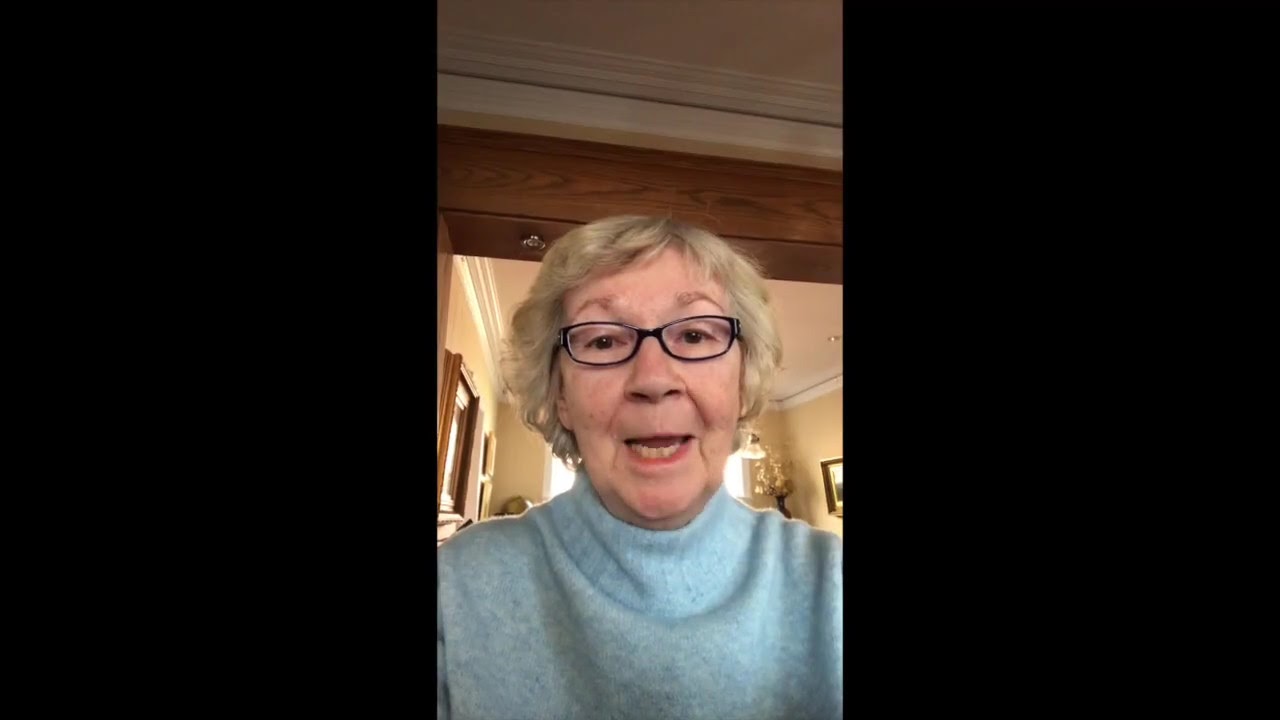A detailed photograph shows an older woman, likely in her 60s, captured mid-sentence during what appears to be a FaceTime or video call. She has short, blonde hair mixed with some graying strands, and she wears black-framed glasses. Her mouth is open, revealing slightly golden-tinted teeth. She is dressed in a light blue turtleneck sweater. The room behind her is painted in a light tan or beige color and features wooden elements, including a brown wooden door frame. The ceiling above is white, and natural light streams in through a window, illuminating the space. Additionally, the background includes framed pictures, a chandelier, a vase with some kind of tree or plant, and a lamp. The image is bordered by black on both the left and right sides, which suggests it may be a screenshot from a video call.